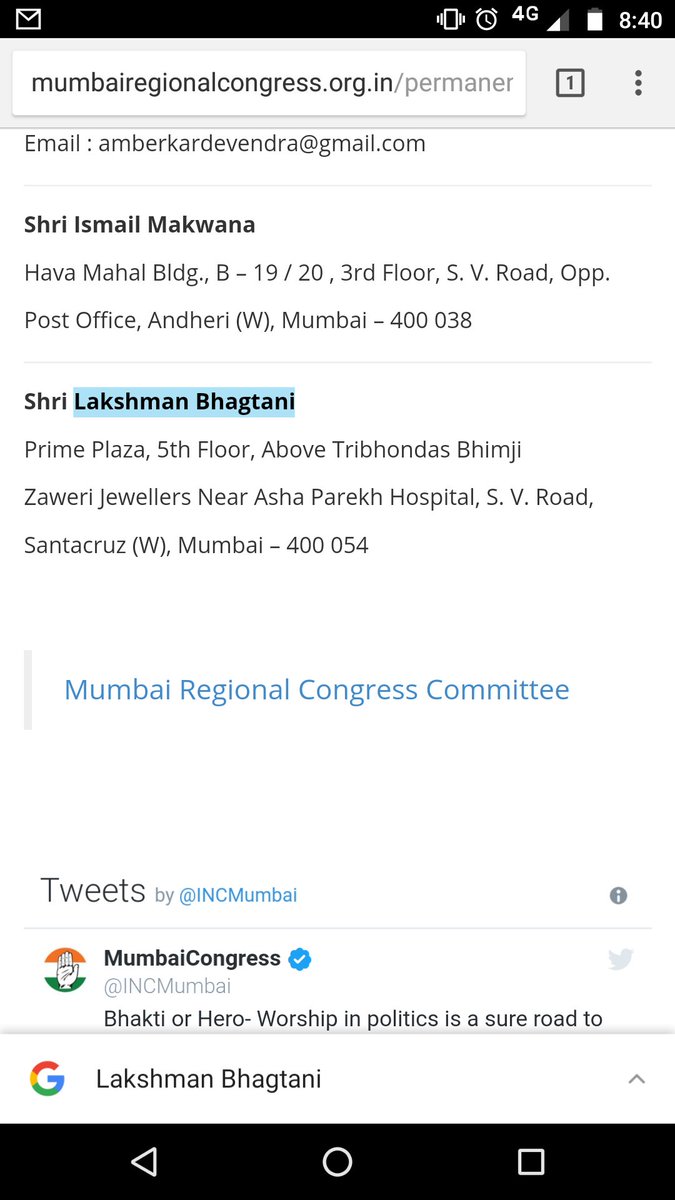The image depicts a smartphone screen showcasing an app, likely a web-based email application or potentially a browser.

At the top, a search box is populated with the URL "mumbairaregionalcongress.org.in/permenir," although the full address is truncated. Below this, an email address is visible: "amberkardavendra@gmail.com."

The content displayed seems to detail contacts or entries related to the Mumbai Regional Congress Committee. The first entry has a header labeled "Sheree Ismail Makwana," followed by an address: "Hava Mahal Building B/1920 Third Floor, SV Road, Opp. Post Office, Indiri W, Mumbai - 400 038."

Further down, another contact, "Shri Lakshman Bhaktani," is listed with the address: "Prime Plaza, Fifth Floor, Above Tribondas Bhimji Zaveri Jewelers, Near Ashwa Pareki Hospital, SV Road, Santa Cruz W, Mumbai - 400 054."

Beneath this, in bold blue text, the phrase "Mumbai Regional Congress Committee" appears, indicating an official connection to the organization.

Towards the bottom, there is a segment featuring a Twitter handle: "Tweets by @INCMumbai." This section includes the Mumbai Congress's verified Twitter account, symbolized by a blue checkmark. Their logo, a stylized depiction of the Indian tricolor flag with an upward-reaching hand, is visible. Below it, a truncated quote begins with "Bhakti or hero worship in politics is a sure road to..."

Lastly, the name "Lakshman Bhaktani" is repeated, accompanied by a Google "G" icon. Standard navigation symbols—a home icon, a back arrow, and a tab button—are present at the bottom of the screen, suggesting typical smartphone interface elements.